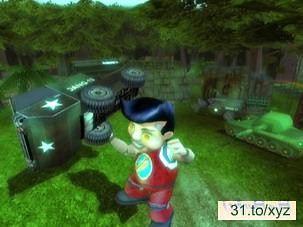In this animated scene, which could depict a video game setting, we observe a dynamic and action-packed moment featuring a central character. The character is dressed in black shoes and a red suit, distinguished by a circle with light blue lighting on the front of his shirt. He has black hair and is striking a powerful pose with his right fist raised in the air, while his left hand appears to have just flipped a nearby army truck. The truck, positioned to the left of the character, is black and green with white stars, now overturned. On the right-hand side of the scene, we see a green tank with its barrel aimed directly at the character. 

At the bottom right corner of the image, there is text contained within a white rectangle, displaying "31.T0.X.Y.Z" in green letters. The ground is covered entirely with vibrant green grass, adding to the vividness of the scene. The background exudes cemetery-like vibes, enhancing the somber atmosphere, and is accentuated by lush green trees with glimpses of blue sky peeking through at the top of the image.